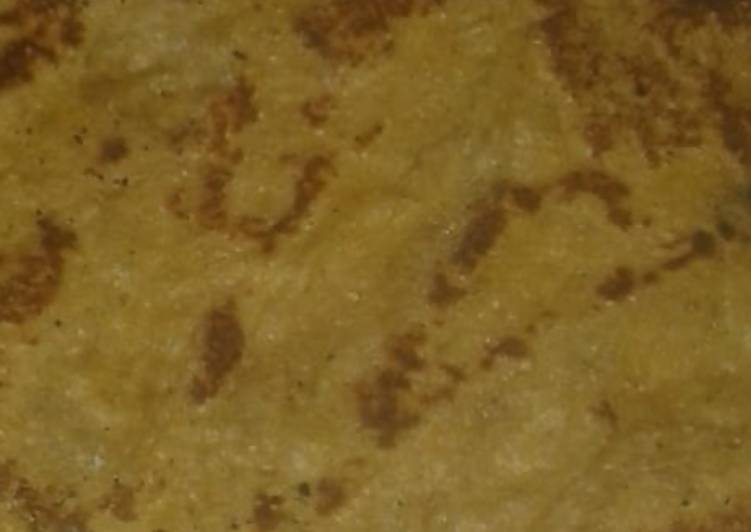In the image, a very zoomed-in view reveals an object that occupies the entirety of the frame, making it difficult to ascertain its precise nature. The object has a light tannish-yellow hue with scattered darker spots, some of which are shaped in distinct forms like a U. The speckles and lines of darker brown are irregularly scattered across the surface, and there is a slight glimmer of oil or moisture visible. The texture is uneven, suggesting it might be a type of food item, possibly a pancake, omelette, or tortilla. This could also be a close-up of a kitchen countertop due to the pattern and texture. The photograph is centered on the object and appears to be of a low quality, lacking any text. The setting might be a kitchen or restaurant, given the context clues and appearance of the object.